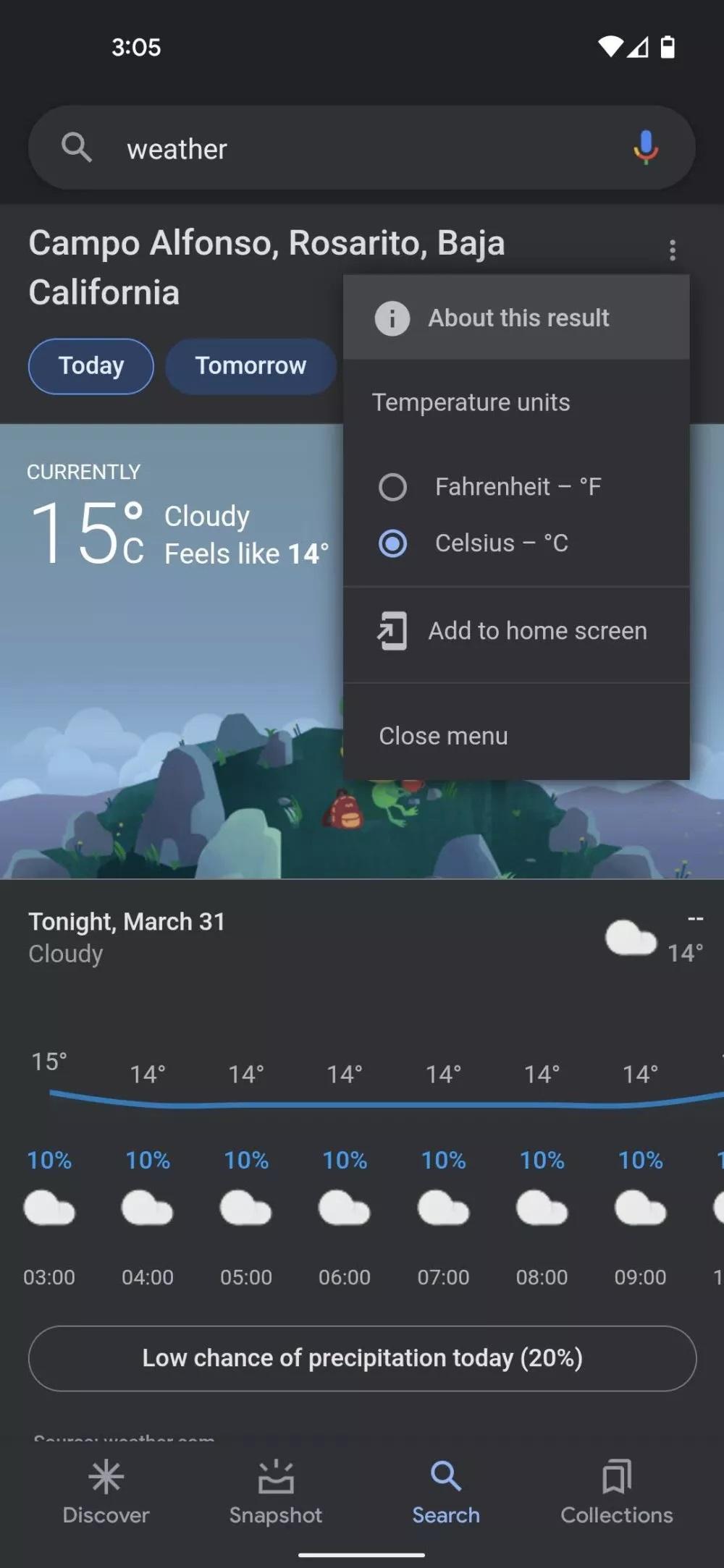The image depicts a home screen displaying a detailed weather forecast for Camp Alfonso Rosarito, Baja California. The time is 3:05, and the battery is nearly full. A search bar at the top shows "weather" as the query. Below, the results for "Camp Alfonso Rosarito, Baja California, today and tomorrow" are presented, with additional options including "About this result" with an information icon, and "Temperature units" where Celsius is selected. 

The current temperature is shown as 15 degrees Celsius, with cloudy conditions making it feel like 14 degrees. The forecast for tonight, March 31st, includes a 10% chance of clouds throughout the hours of 3 PM to 9 PM. Additionally, there's a low 20% chance of precipitation today.

At the bottom, there are navigation options for "Discover" (marked with a star), "Snapshot," "Search" (represented by an hourglass), and "Collections" (depicted as a file folder). Overall, the screen provides a comprehensive weather overview for the specified location in California, including current temperatures, cloud cover predictions, and chances of precipitation, all within a user-friendly interface on a browser application.